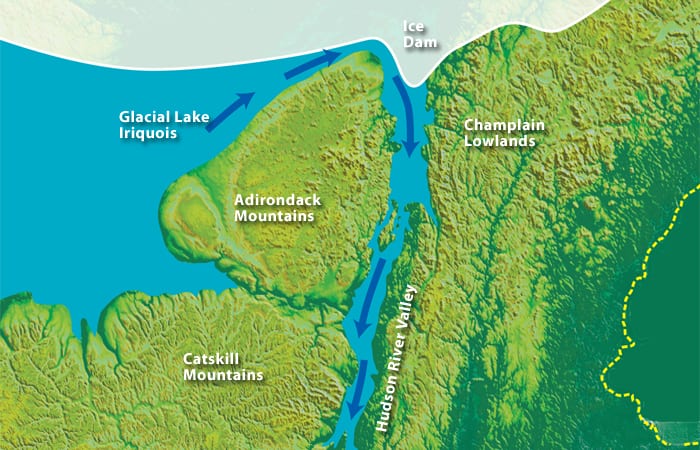The image is a horizontally aligned rectangular map and diagram illustrating topographical features and ice movements. At the top, a curved gray section labeled "Ice Dam" in white text indicates a significant glacial feature. Below, the upper left section showcases a solid blue area labeled "Glacial Lake Iroquois," from which blue arrows indicate water flow, angling upward to the right and then descending vertically through the map's center.

Surrounding the central waterways are various landmasses. The right side features the "Champlain Lowlands," shaded primarily in light green with a significant portion in dark green, which also contains a dashed yellow line. The label "Hudson River Valley" is prominent in this region as well. On the left side, the map depicts the "Adirondack Mountains" above and the "Catskill Mountains" below, both shaded in a similar light green with darker green borders. The map’s topography is depicted through varying shades of green and shadowing to illustrate elevation and terrain differences.

Overall, this detailed diagram effectively portrays geological and glacial interactions, emphasizing key regions such as the Champlain Lowlands, Hudson River Valley, Adirondack Mountains, Catskill Mountains, and the historical extent of Glacial Lake Iroquois.